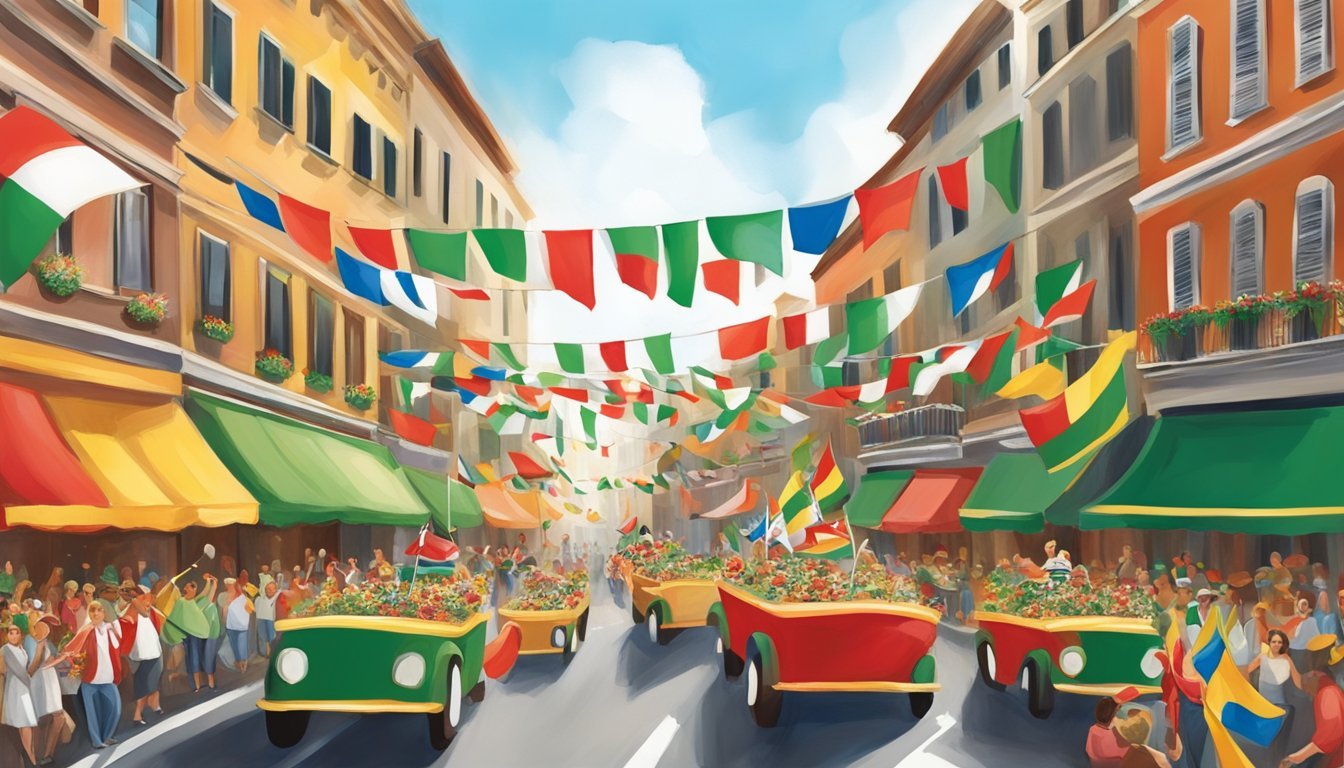The painting depicts a vibrant, celebratory parade scene on a wide, paved road flanked by tall, colorful buildings. The parade features an array of unusual open-topped vehicles, resembling wagons or box-like cars, in vibrant colors of green, yellow, and red. These vehicles are packed with cheerful people and decorated with flowers, moving down the street without any visible means of propulsion. The scene is adorned with an abundance of flags stretched across the street from building to building, creating a festive atmosphere. These flags, in hues of red, green, blue, white, and black, contribute to the lively and colorful aesthetic of the painting. The buildings lining the street are a mix of apricot, gray, yellow, beige, and orange, with multicolored awnings and some having plants outside their windows. The foreground is filled with a dense crowd of spectators on both sides of the street, all depicted in a simplified, almost childlike style, adding to the painting’s primitive and whimsical charm. The sky above is a bright blue with scattered clouds, enhancing the scene’s cheerful and celebratory vibe, and the image compositionally stretches out more in length than in height.